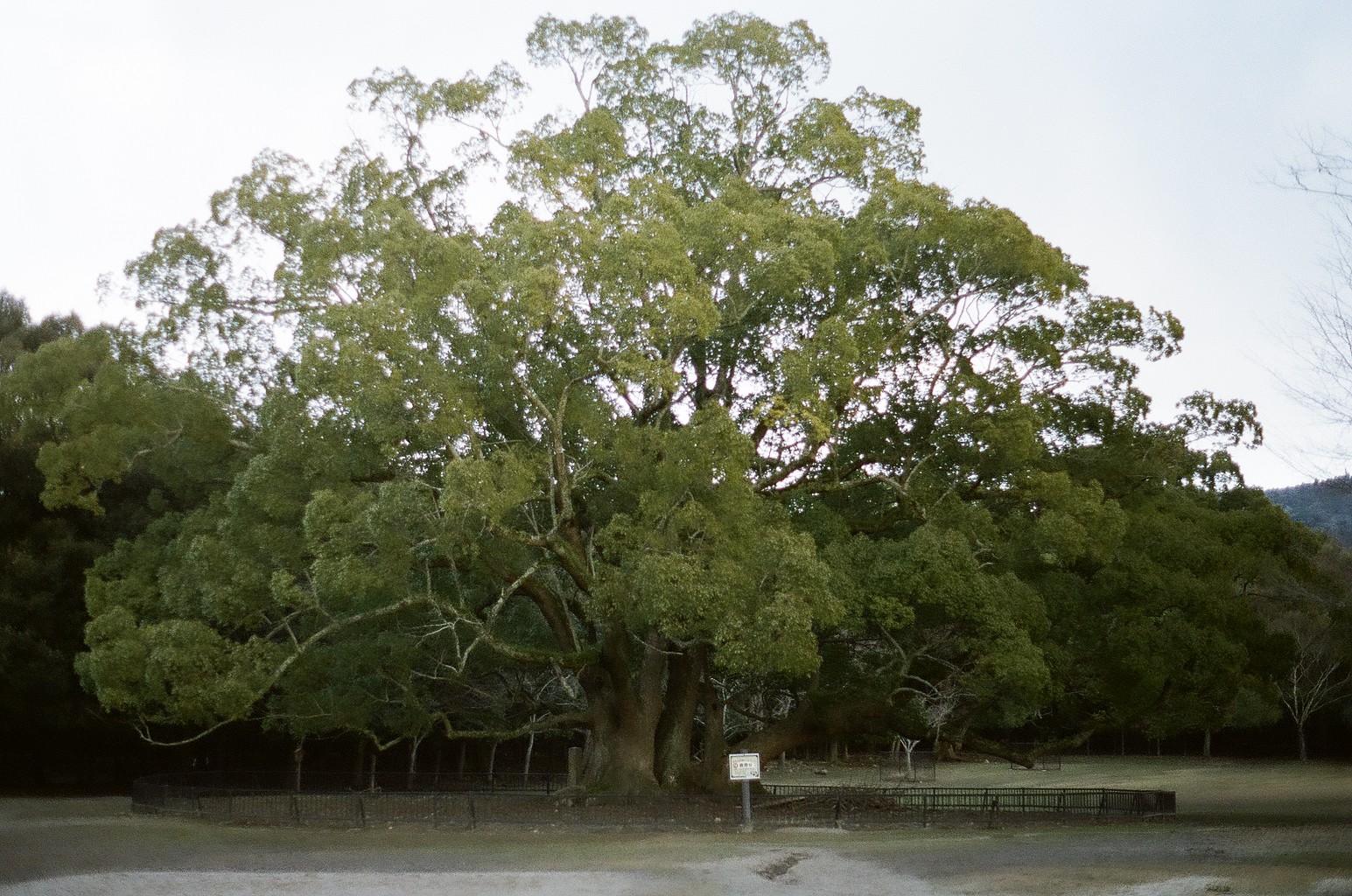This horizontal rectangular photograph captures a serene natural scene dominated by an imposing and unusually wide tree. The tree is noteworthy due to its expansive trunk, which bifurcates into five or six large sections at the base, giving it a grand, dominating presence in the center of the image. Its dark brown trunk and branches support a lush, green canopy, emphasizing its prominence in the landscape. In front of this massive tree stands a small white sign mounted on a post, though the text on the sign is unreadable due to its distance from the camera. Surrounding the tree is a mix of stone surfaces and a brownish river, flowing from one side of the image to the other, with rocks lining either side of the water. Behind the central tree, a dense bank of other trees stretches across the background, under a uniformly cloudy sky which casts a soft, diffuse light over the entire scene. There are no people or vehicles visible, highlighting the tranquility and untouched nature of the setting. The area is fenced, suggesting the significance or protected status of the large tree.